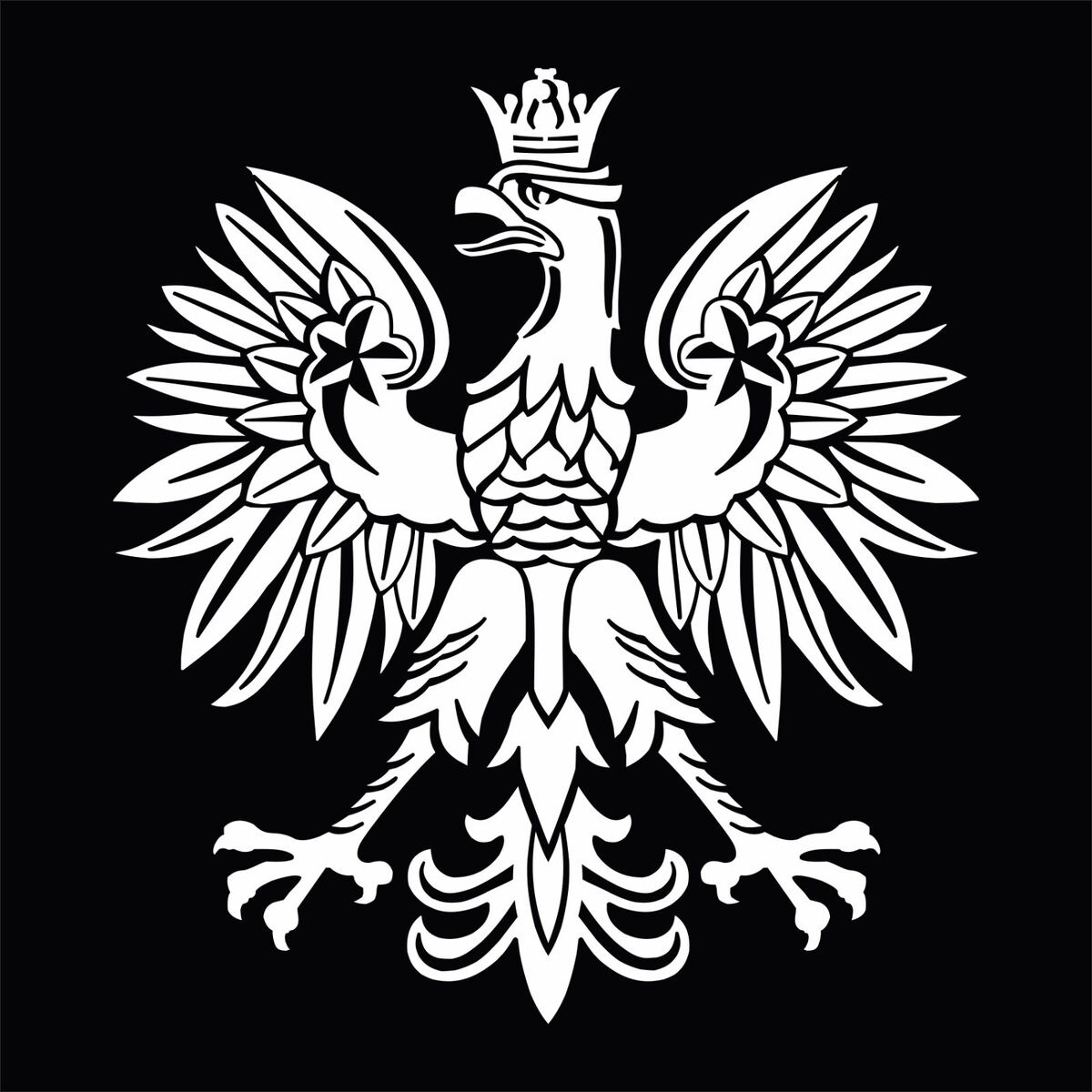The image is a detailed black and white pen and ink drawing set against a solid black background. It features a large, majestic eagle prominently positioned in the center, exuding a regal presence with its striking pose and intricate details. The eagle's legs are apart in a straddle position, showcasing four sharp, expanded claws on its feet. Its impressive wings are outstretched to the sides, forming a wide, graceful arc. The bird's head is turned to the right, displaying its profile crowned with a delicate royal crown. The wings are adorned with two stars, adding to the ornamental design. The eagle's feathers are meticulously detailed, with those on the torso resembling scales, contributing to the texture and depth of the illustration. Its tail feathers are particularly ornate, extending outward in a crescent-like shape. This intricate depiction captures the grandeur and authority of the eagle, making it a powerful and emblematic symbol against the stark black background.